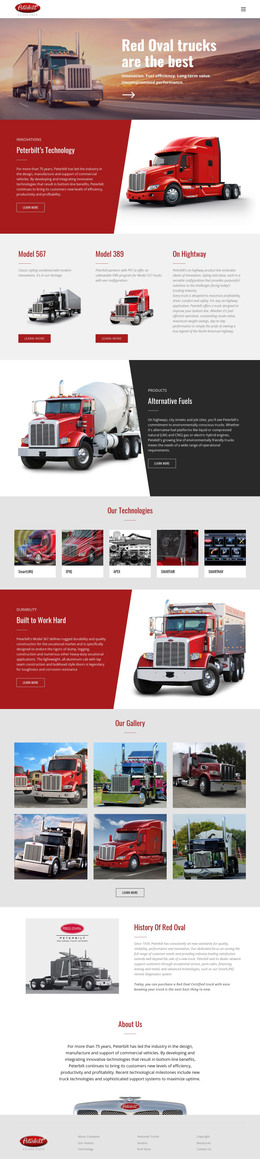The image depicts an informational page about tractor-trailer trucks with a prominent header at the top stating "Red Oval Trucks are the Best." The header features an image of a tractor-trailer. Below the header, on the right, is another red tractor-trailer, and adjacent to it on the left is a red section with text that is too small to read. Underneath this, there is a white section divided into three parts, each containing text. The first two parts feature images of different tractor-trailers with their names written in red, although the text is too small to decipher. 

Following this, there is a section with a cement mixer on the left, which has a red cab and a white mixer, and to the right of it, a black section presumably containing information about the cement mixer truck. The next segment is a gray area showcasing five truck images, each labeled underneath. Another section, similar to the top one, features a red text block on the left and an image of a large truck to the right.

Further down, there are six truck images, and at the bottom of the page, there are three sections. The first section includes a truck image, the second contains text, and the third likely provides information about the company, indicated by the words "About Us."